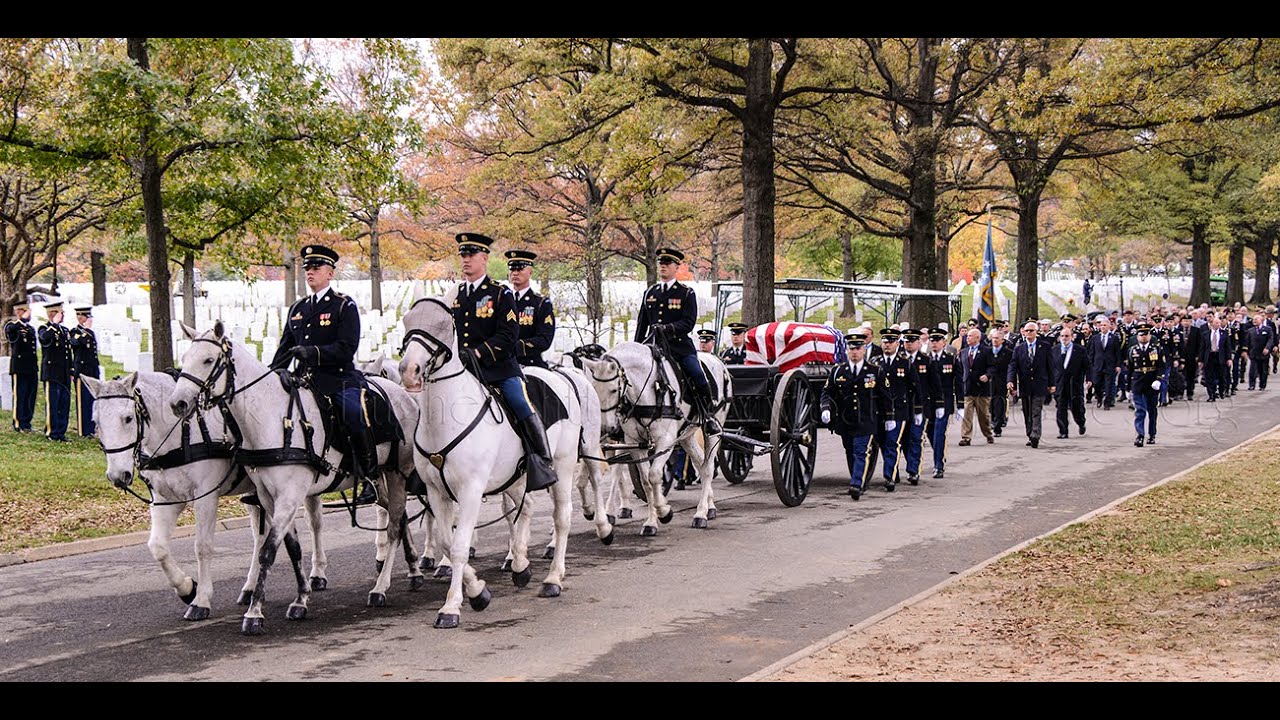This color photograph captures an elaborate U.S. military veteran's funeral procession on a gray asphalt road, flanked by light green foliage and trees in the background. Leading the solemn event are white horses with black harnesses and hooves, ridden by four men adorned in navy blue military uniforms bearing military insignia, and black and gold military hats. The horses are pulling a black wooden wagon that carries a casket draped in a red, white, and blue American flag, with the red and white stripes and blue starred field distinctly visible.

Flanking either side of the wagon are numerous military personnel, walking in the same navy blue uniforms as the riders. As the procession advances, it's followed by a larger crowd consisting of more military officers and civilians dressed in suits. To the back left, a graveyard is partially visible, further reinforcing the somber, respectful atmosphere of this final tribute. In the background, additional soldiers stand in attention, saluting in their military attire.